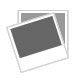The image is the cover of a program or guide, likely handed out during a professional soccer match. The top of this magazine features a red horizontal bar with the word "STADION" in bold white capital letters, and "AKTUELL" in thin black lowercase letters beside it. To the right of the title, there is a white shield logo with red letters at the top, which includes the name "STUTTGART" and a yellow inverted triangle within the logo. 

The cover prominently displays a soccer player in a white uniform with a red horizontal stripe, white socks with red stripes at the top, and white shoes. The player, who has short black hair, is captured in motion, running with his right hand placed across his heart and his left arm extended behind him. In the background, two players in blue uniforms from the opposing team are visible on the green grass pitch. Additionally, spectators can be seen in the stands, as well as various sponsor logos.

The text indicates dates and names possibly relevant to the match, such as "4-10-2008," "SV Werder Bremen," and mentions of various competitions including the "Bundesliga" and "UEFA Cup 1 Haupttrund." The language appears to be German, suggested by the references to Stuttgart and possibly German football terminology.